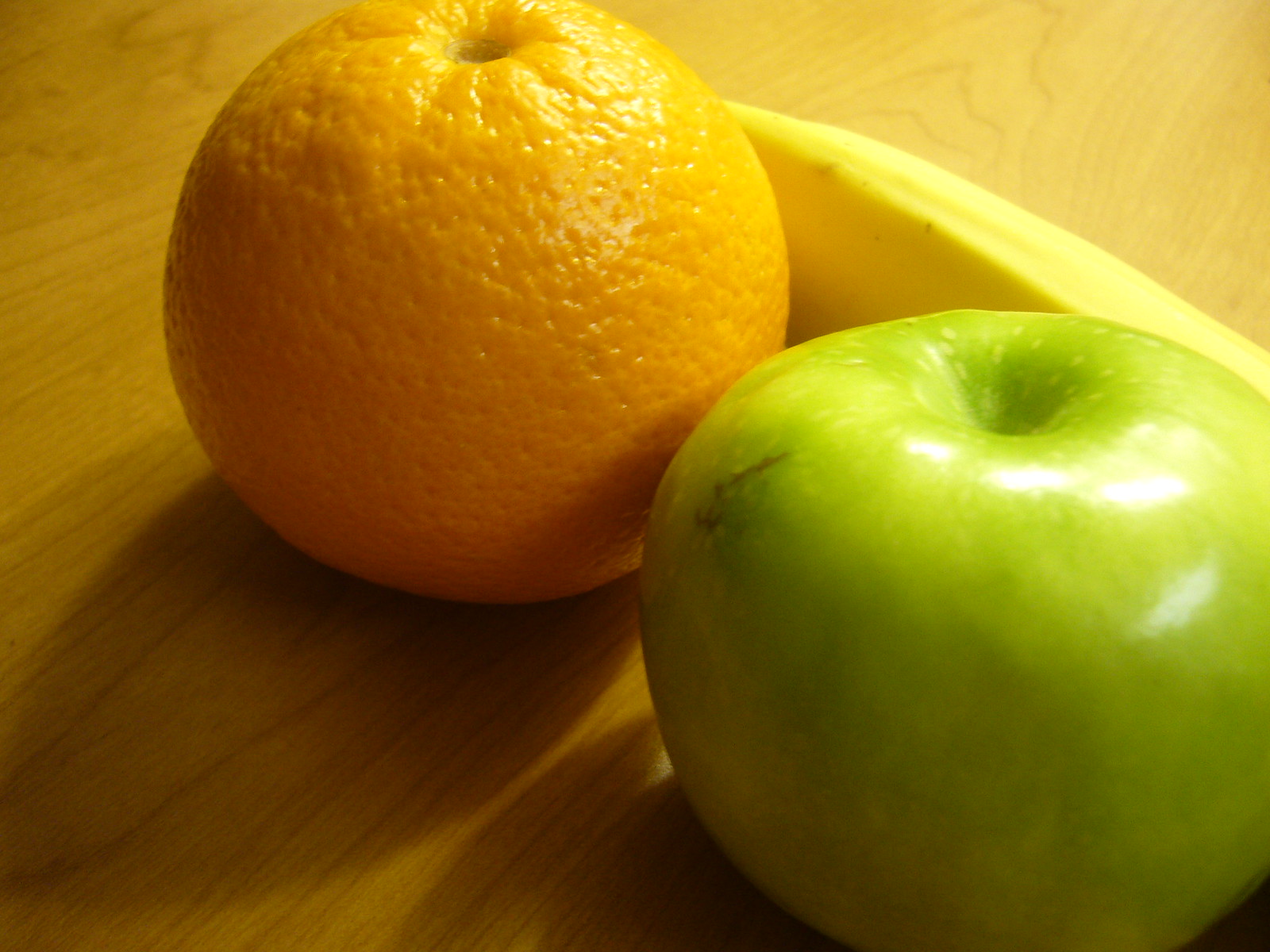This close-up image captures a slightly angled view of a collection of fruits laid out on a wooden surface. The table appears to be made of unadorned honey-yellow wood, characterized by visible grain patterns and subtle shadows that play across its surface, suggesting a basic, functional design rather than a decorative one. No specific background details reveal the location, leaving it ambiguous whether the setting is a kitchen or some other place. 

In the bottom right corner, a green apple takes center stage with patches of light reflecting off its shiny surface, and a small, distinguishable blemish marring its otherwise smooth exterior. Adjacent to the apple, there is a wrinkly clementine, exuding a rustic charm with its textured peel. Just behind the clementine, a glimpse of a yellow banana peeks into the frame, adding a splash of brightness to the ensemble. The natural interplay of light and shadows accentuates the colors and textures of the fruits, creating a visually appealing and intimate portrayal of these everyday items.